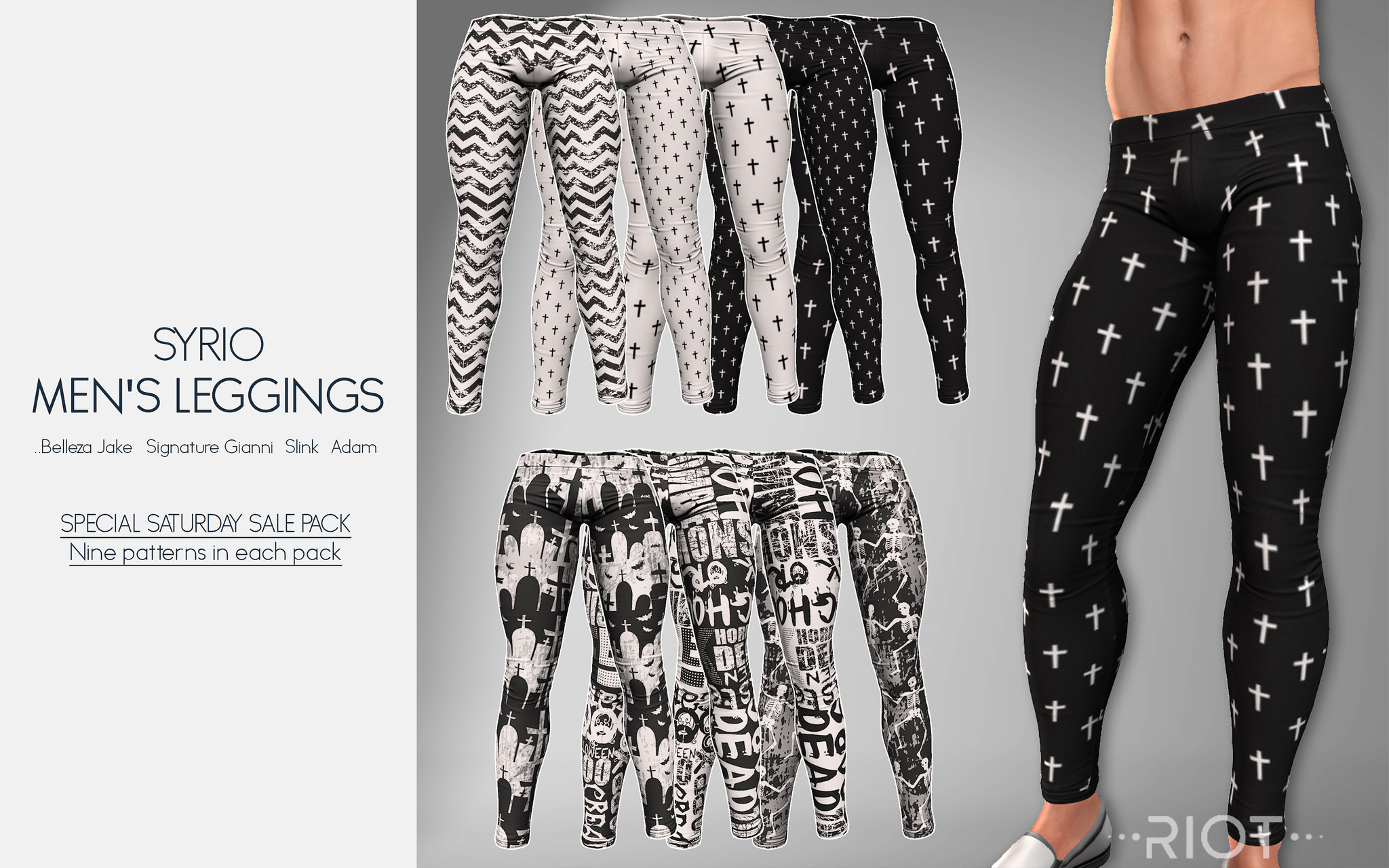The image is an advertisement for men's leggings branded as Cyreal Men's Leggings. On the far left of the image, a grey background displays text listing various styles: Basilia, Jake, Signature, Gianni, Slink, and Adam. Below this, it reads "Special Saturday Sale Pack" and notes that there are "Nine Patterns in each pack." The ad showcases leggings in various black, white, and grey patterns, including designs with black and white crosses, zebra lines, and text slogans. Positioned on the right side of the ad, there's the lower half of a model's body, from just above the navel down to the feet, showcasing the leggings. This model is wearing a pair of black leggings adorned with white crosses, complemented by white bedroom slippers. The model’s skin tone is light, and the leggings fit tightly, highlighting the detailed patterns and the snug fit of the product.